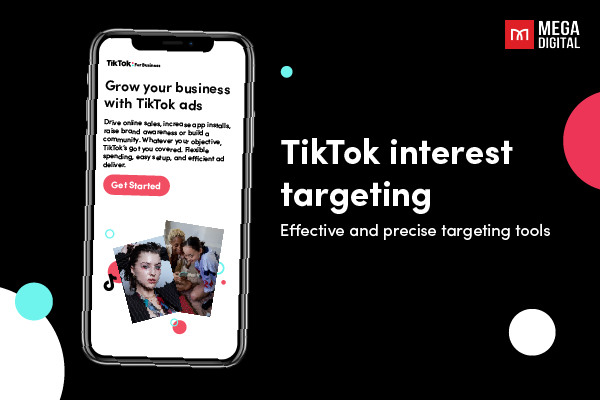This image features a section of a website primarily showcasing an advertisement banner. In the top right corner, bold white text proudly displays "Mega Digital." To the left of this text, a vibrant red square frames a prominent letter "M" in the center. The background of the banner itself is a sleek black, giving the entire section a modern look.

On the bottom left of this black background, there is a partially visible white circle with a smaller light blue circle positioned on top of it. Nearby, a small white circle sits to the right of this feature. Towards the top right is the visible half of a red circle, with an additional very small light blue circle situated centrally at the top.

To the left of this blue circle, a stylized cell phone icon is present. Directly adjacent to this is a compelling promotional message in white text: "Grow your business with TikTok ads." Beneath this headline, a concise paragraph in black text elaborates on this opportunity. Below the paragraph lies a striking red button labeled "Get Started."

At the bottom right of the ad, white text reads, "TikTok interest targeting: Effective and precise targeting tools." This tagline reinforces the focus on TikTok's advertising capabilities, aiming to attract business owners to leverage the platform’s specialized marketing tools.

Two small photographs of people are positioned near the red "Get Started" button, likely adding a personal touch or testimonial element to the advertisement. The detailed and thoughtfully arranged elements from top to bottom, and side to side, create a visually compelling and informative ad display.